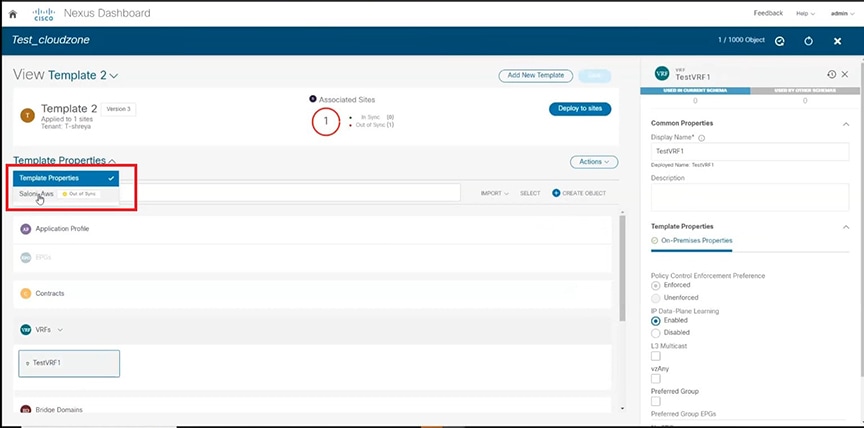**Detailed Caption: Cisco Nexus Dashboard Screenshot**

The screenshot showcases a Cisco Nexus dashboard, specifically designed for router configuration. Dominating the top of the interface, a blue bar prominently displays the text "test_cloud_zone." On the far right of this bar, there are indicators showing "1 of 1 / 1000 objects," followed by a check mark, an "X" icon, and a power button symbol.

Directly above the blue bar, a navigation menu offers several options including "Menu," "Feedback," "Help" with a dropdown menu, and "Admins" also featuring a dropdown menu. Further interface elements include a "View in black" option and "Template 2" highlighted in blue with a collapsible menu. 

The details of "Template 2" reveal that it is applied to one site's tenant in a T-shared area, version 3. An indicator shows associated sites marked with a circled "1," specifying "In sync: 0" and "Out of sync: 1." A blue button with white text reads "Deployed to sites."

Below this, there are various template properties encapsulated in a red outline. "Saloni AWS" is partially visible, indicating the involvement of AWS configurations. Adjacent options include dropdown menus for importing, selecting, and creating objects, signified by a plus mark. Additional features include an "Actions" dropdown menu, "Application Profile Option," "EPG," "Contacts," "VRFs," and a specific "Test VRF1" with its own dropdown menu. 

Towards the bottom right, there is an option labeled "Bridge Domains." On the right side of the screenshot, detailed common properties such as "TZRF1," alongside descriptions of template properties, are visible. Settings include "Poly Controlled Force Preference" with "Enforced" and "Unenforced" as available options, with "Unenforced" currently checked. Other configurable details include "IP Data Learning," multicast settings, and preferred group EPG settings. 

The intricate details and various options clearly indicate that the dashboard is designed for advanced router and network configurations, emphasizing its utility for IT professionals managing complex networking environments.